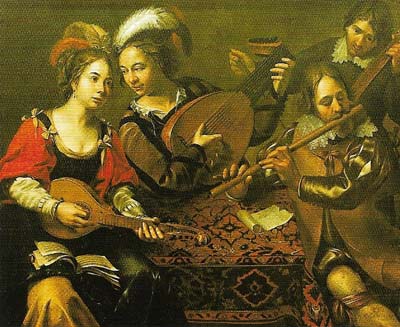This painting, steeped in an old-fashioned and medieval aesthetic, portrays a quartet of musicians gathered around a table draped with an intricately detailed carpet-like tablecloth in shades of brown and black. On the left, a woman plays a banjo or similar stringed instrument, adorned in a vibrant red-sleeved dress with a black bodice and a distinctive feather in her hair tied back in a loose bun. Beside her, another woman, similarly adorned with a white feather, engages with a comparable stringed instrument. Her attire features brown sleeves against a darker central garment. To her right, a man, deeply immersed with closed eyes, plays a wooden flute, dressed in a gold shirt under a gold-tinged coat, exuding a sense of motion. Above him, another man, depicted in a blue shirt with white collars and brown hair, handles a large stringed instrument, possibly a cello, contributing to the harmonious scene. The group is set against a dark green background, enhancing the timeless feel of this evocative painting.